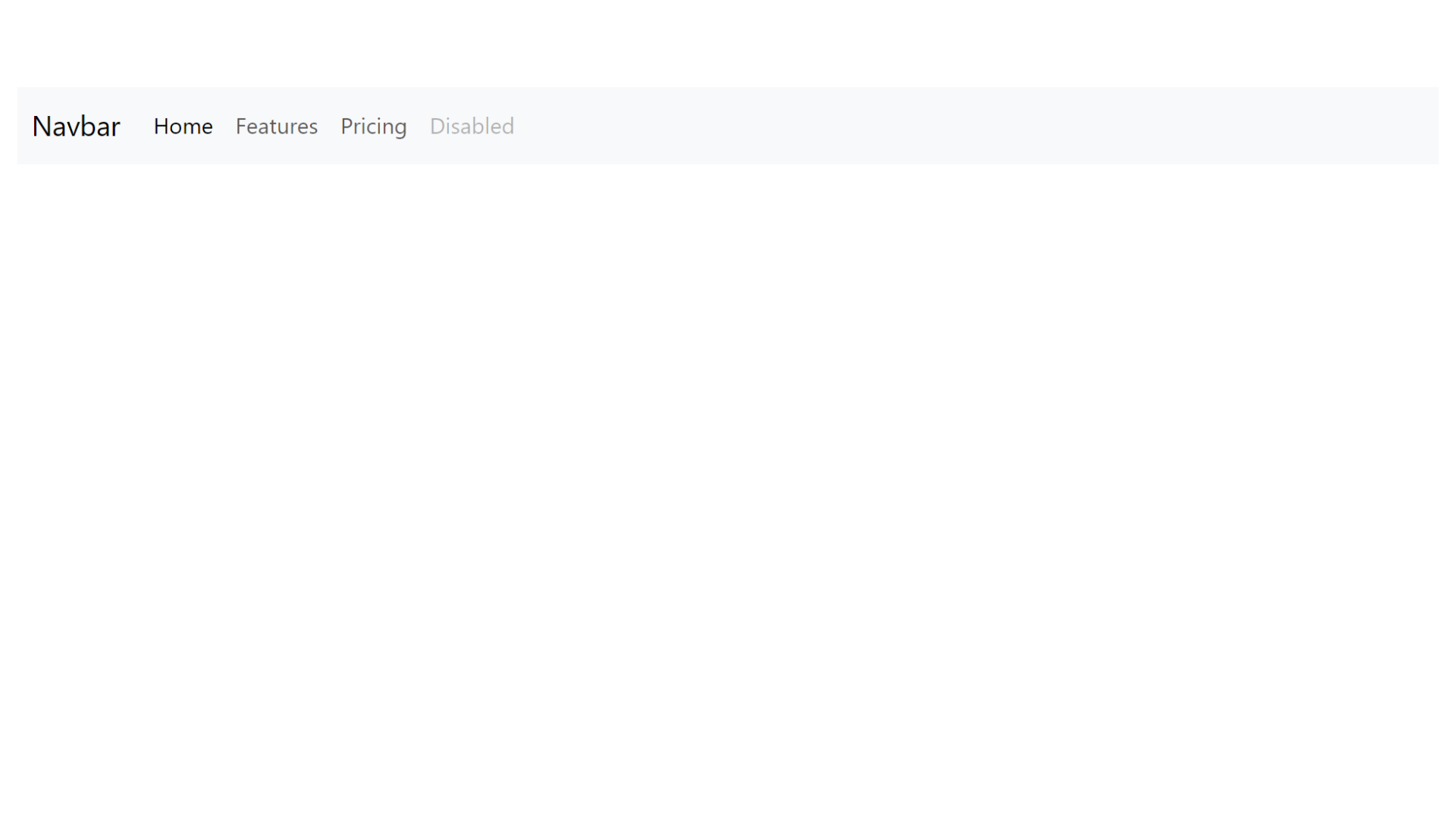The image captures a minimalist navigation bar set against a plain white background. The navigation bar itself is gray and spans horizontally across the top of the image. At the leftmost section of the bar, the word 'Navbar' is displayed in black text with the 'N' capitalized, while the rest of the letters are in lowercase. 

Moving rightward within the bar, there is a label that reads 'Home', with the 'H' capitalized and the subsequent letters in lowercase. Continuing along, a small gap leads to the word 'Features', where only the 'F' is capitalized. 

Further to the right, another space separates 'Pricing', again formatted with just the 'P' capitalized. Finally, at the far right of the navigation bar, the word 'Disabled' appears in a much lighter gray, making it less prominent compared to the other labels. The text progressively lightens from left to right, with 'Navbar' and 'Home' being the most visible, while 'Disabled' fades into a subtler shade.